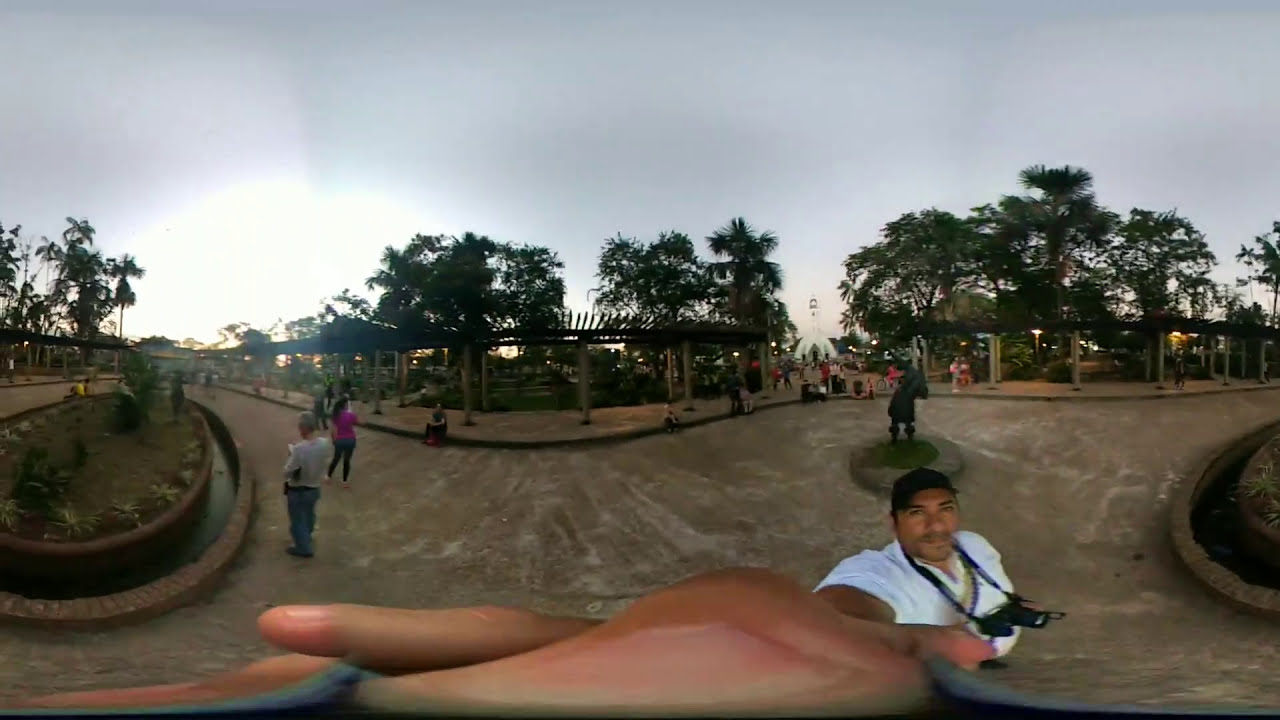This photo, slightly distorted towards the bottom, appears to be of a resort-like area shot in a spliced, 360-degree selfie style, creating a warped view. It depicts a man in a white shirt with a black camera around his neck, possibly holding a selfie stick. The ground beneath him is tan-colored, resembling a terracotta or brick surface, not typical asphalt. The surroundings feature abundant greenery with trees and shrubs, as well as large round terracotta planters. There are numerous people, likely tourists, ambling along the pathway that extends through what seems to be the entryway of a park or recreational area, possibly in a tropical setting. The sky above is mostly cloudy, casting a subdued light over the scene with some walkway lights starting to illuminate. The colors present in the image include shades of blue, gray, white, green, brown, purple, pink, tan, and more, giving it a vibrant yet scattered appearance.